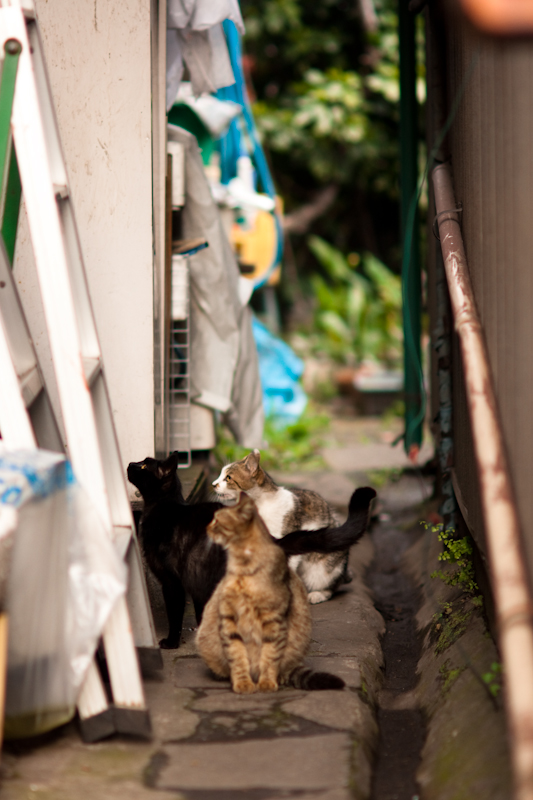In a cluttered, narrow alleyway, framed by a brown wall on the right and the white side of a slanted building on the left, three cats command attention. This cramped space, barely wide enough for a person to navigate, is decorated with a scattering of household items: a white ladder leaning against the left wall, plastic bags, blue fabric hanging from the walls, and an air conditioning unit. A light brown tube snakes its way across the center of the scene. At the end of this four to five-foot-long alley lies a blurred backdrop of plants and a fence.

The main subjects, three cats, sit intently looking up to the left. Closest to the viewer is a brown tabby cat, marked with dark stripes. Next to it is a black cat, and slightly behind them is a white cat adorned with brown and gold splotches. Their collective gaze is fixed on the ladder or possibly an open window, suggesting something of interest or curiosity has captured their attention. These well-fed felines present their heads in profile, creating a compelling scene of anticipation and alertness amidst the everyday alleyway chaos.